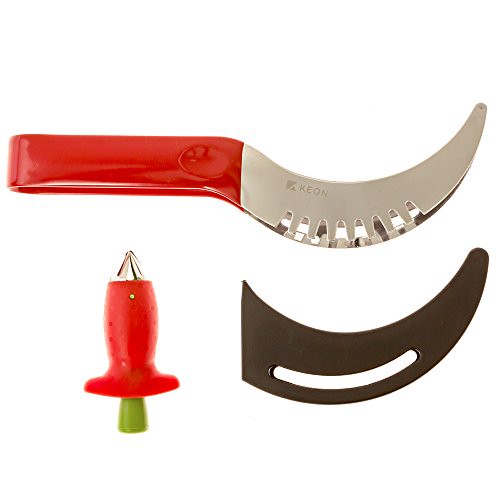The image is a professional advertising photograph with a white background, featuring three distinct kitchen utensils. The top utensil is a unique knife with a horizontal bright red handle and a curved stainless steel blade, forming a C shape. The blade also features light gray text that spells "KEON." Below this knife, to the left, there is another object resembling a vertical plug or topper. Its base is a blue rectangle, transitioning into a plunger shape that is wide at the bottom, narrows in the middle, and has a stainless steel pointed tip at the top, suggesting a fruit corer. Adjacent to this, on the bottom right, is a black plastic knife guard designed to protect the curved blade. This guard has a slit that resembles a smile, fitting the shape of the knife blade perfectly. Together, these utensils appear to be specialized tools for fruit preparation and cutting.